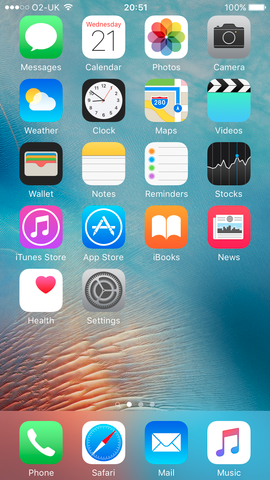The image showcases a detailed screenshot of an Apple iPhone home screen, featuring an assortment of app icons and status indicators.

At the top-left corner, a green square icon with a white chat bubble represents the messaging app, while next to it an orange calendar icon signifies "Wednesday 21". Adjacent to the calendar icon is the vibrant "Photos" app, displaying a colorful pinwheel in shades of red, purple, blue, green, yellow, and orange. Continuing to the right, the "Camera" app icon appears as a black camera silhouette, followed by the "Weather" app symbolized by a cloud and sun on a blue background.

The middle row begins with the "Clock" app, shown as a traditional clock face, followed by "Maps," resembling the familiar Google Maps icon. Next to it, the "Videos" app icon features a blue background with an action bar image. The "Wallet" app icon displays various colored cards peeking out of a gray-to-black wallet graphic. The "Notes" app is represented with an orange header and lined paper design. The "Reminders" icon stands out with four colorful dots—orange, blue, green, and purple—above black lines on a gray background. The "Stocks" app, depicted with a black icon showing a gray graph and blue dot, and the "iTunes Store" with a purple background and white music symbol, are also present. Completing this row, the "App Store" icon features a white "A" inside a blue circle, and "iBooks" is shown with an open white book on an orange backdrop. The "News" app icon looks like a red newspaper, displaying an image of mountains or trees.

On the next row, the "Health" app icon, illustrated as a white square with a red heart, precedes the "Settings" icon, which features a gear on a dark gray background. 

At the bottom dock, the "Phone" app icon, in dark green with a phone receiver image, is positioned next to the "Safari" browser icon, showing a blue compass with white and red tips pointing west and east, respectively. The "Mail" app icon, characterized by a dark blue envelope, and lastly, the "Music" app, boasting a white background with a gradient music note transitioning from purple to red to dark blue, which is set against a visually dynamic wave pattern in blue, orange, and pink, frame the dock icons.

Status indicators across the top bar reveal full cellular signal strength (three dots) next to the O2-UK carrier symbol. This is followed by a full wireless signal symbol, the time displayed in military format (20:51), and the battery level at 100%.